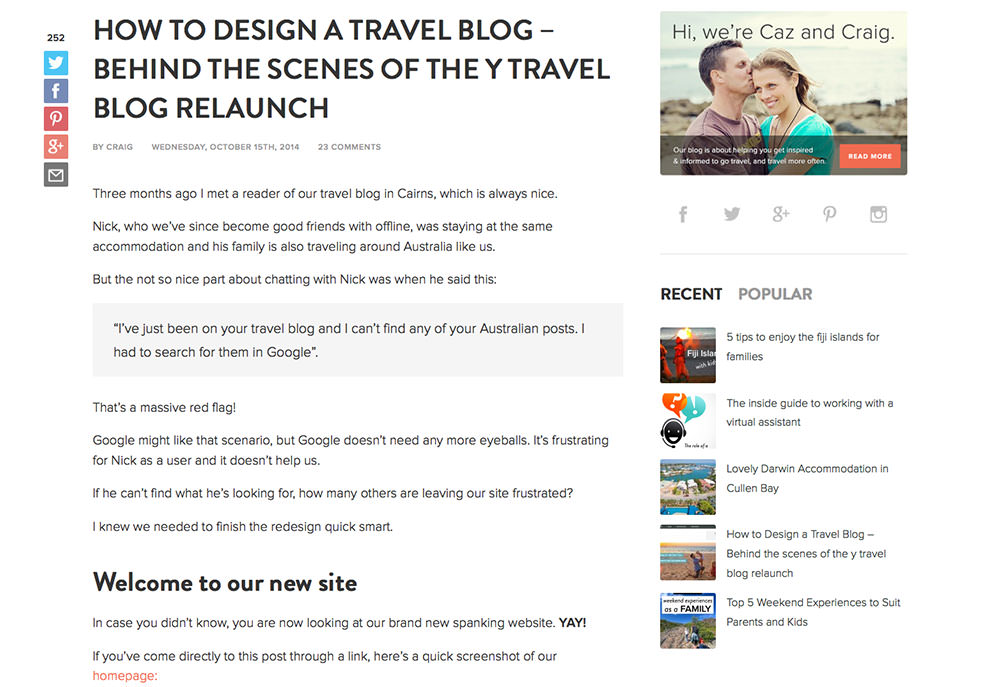In large, bold black letters at the top, the image displays the title "How to Design a Travel Blog: Behind the Scene of the Why Travel Blog Relaunch." On the left, the number "252" is followed by icons for Twitter, Facebook, Pinterest, Google Plus, and an envelope icon. Below that, the article is titled "By Craig," dated Wednesday, October 15, 2014, with 23 comments.

The caption continues with a detailed narrative: "Three months ago, I met a reader of our travel blog, Karen's, named Nick. Meeting readers is always nice, and we have become good friends with Nick both online and offline. Coincidentally, we were staying at the same accommodation, and his family is also traveling around Australia, just like us. However, the not-so-nice part of our conversation was when Nick mentioned, 'I've just been on your travel blog and I can't find any of your Australian posts. I had to search for them on Google.' This feedback was a massive red flag. While Google might appreciate that scenario, it doesn't need more traffic. It's frustrating for Nick as a user, and it certainly doesn't help us."